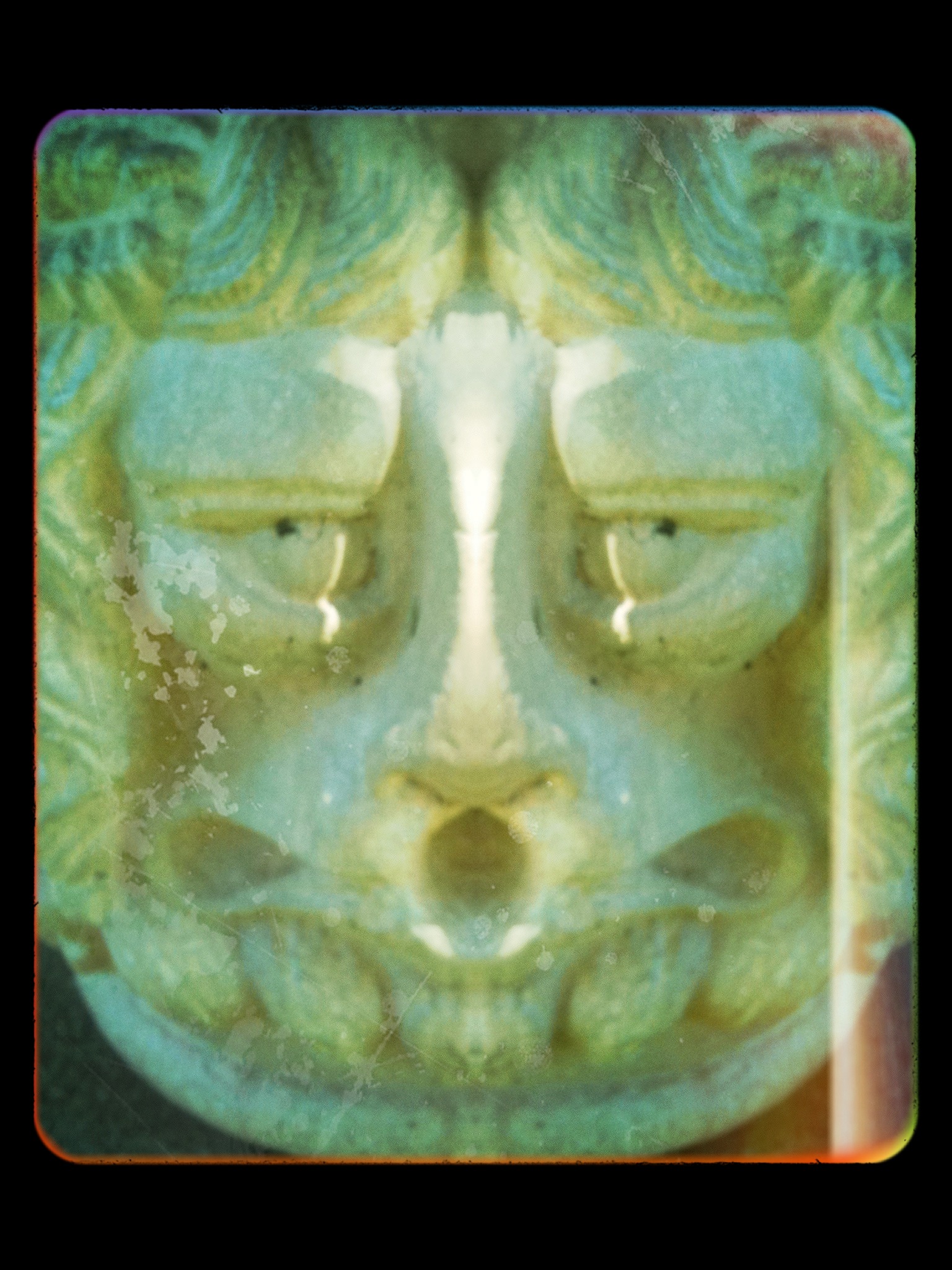The image depicts a close-up of a concrete sculpture framed by a black border. The sculpture appears to be crafted from a white or off-white material and features a vertically rectangular shape. Dominating the center is a disturbingly expressive face with an evil appearance. The face has long, curly hair that surrounds its head, bulging eyes with small pupils, and a prominent nose with additional holes beneath it, giving it an exaggerated and grotesque look. The mouth is slightly open, revealing five large, top teeth. The cheeks also have holes, adding to the eccentric design. The overall composition suggests a symmetrical layout, where dividing the face down the middle would result in mirrored halves. This bizarre and elaborate artwork is likely resting on a table, captured in the photo with great detail, showcasing the eerie and unsettling features of the statue.